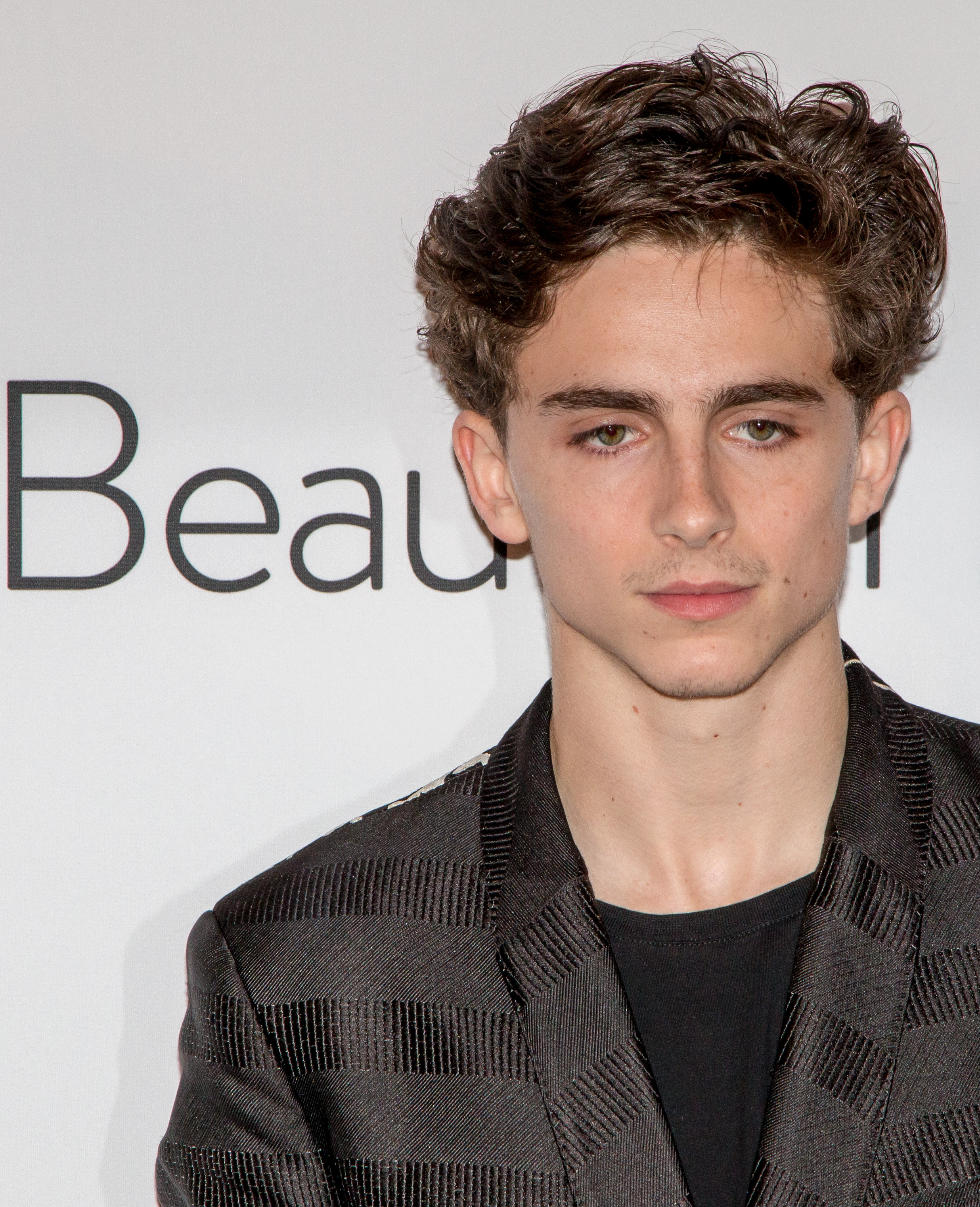The image depicts young actor Timothy Chalamet standing in front of a white wall with black letters partly obscured by his head, spelling out "B-E-A-U." He has short, wavy, and slightly unkempt brown hair, and is clean-shaven with a hint of stubble around his chin and jawline. Chalamet is wearing a stylish black t-shirt paired with a textured, striped black jacket that resembles a suit but isn't smooth. He appears to be staring slightly downward with a neutral expression. The image is very well-lit, clean, sharp, and bright, highlighting every detail clearly.